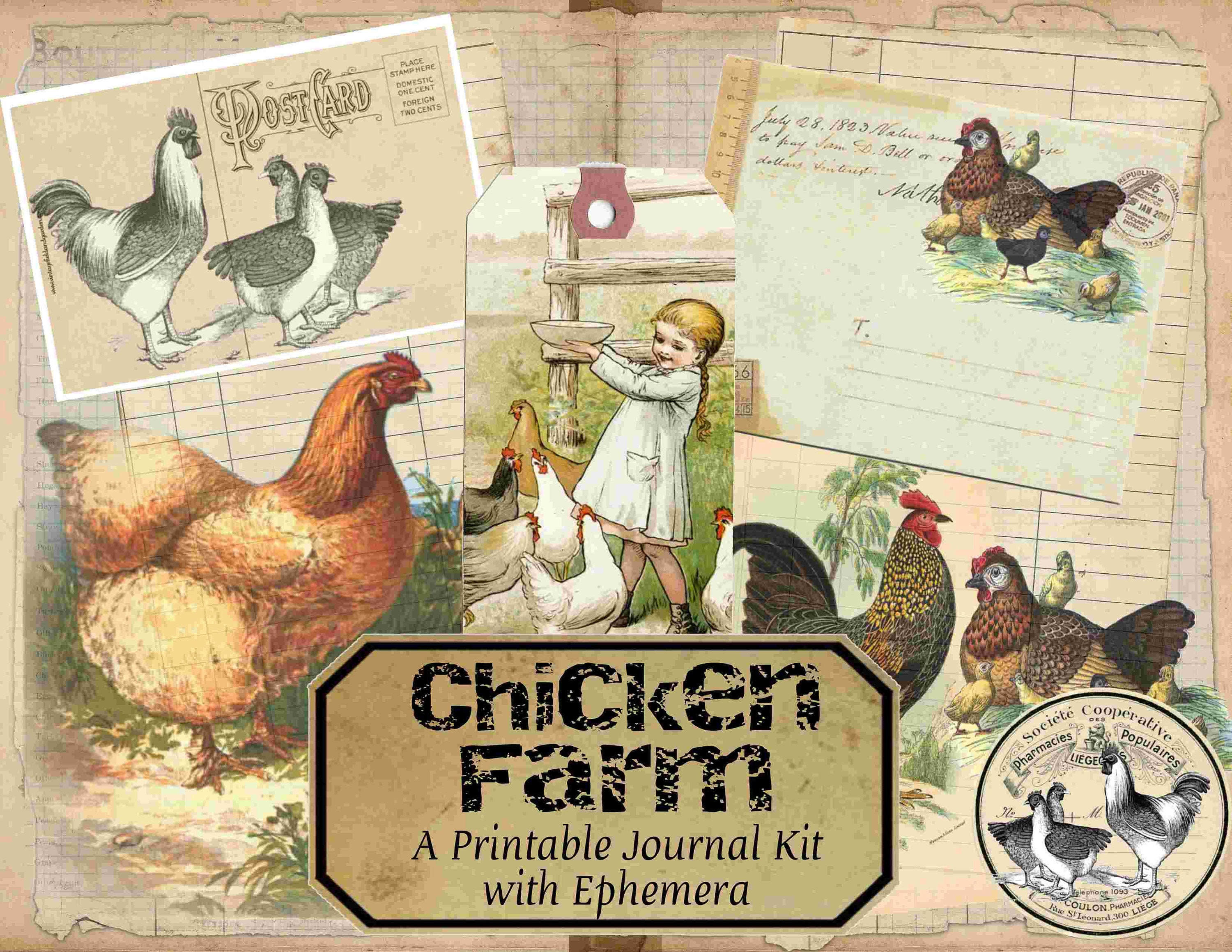This journal kit cover is a captivating collage that tells a story of farm life, centered around chickens and rural imagery. Dominating the cover is a vividly detailed scene featuring several chickens: a prominent large brown chicken on the left, a colorful green and yellow rooster facing a smaller brown hen on the right, and assorted baby chicks scattered around. At the bottom of the cover, a black-bordered, gold plaque displays the title in bold black text: "Chicken Farm - A Printable Journal Kit with Ephemera." 

Interspersed among the chickens are various nostalgic elements. On the top left, there's a black-and-white postcard depicting more chickens. Adjacent to it, a charming photograph shows a young girl in a white dress, holding a bowl in preparation to feed the chickens by a rustic fence. This image is brimming with life as smaller chickens gather around her. 

To the right, the cover features another postcard with a rooster and two chickens. Beneath these, the logo of the Society Cooperative is prominently shown, featuring an illustration of ducks. This logo reappears in a reversed form as a sticker at the bottom, harmonizing with the overall theme. The background is a serene farm scene with wandering chickens, adding to the pastoral ambiance.

All these elements collectively create a richly textured and nostalgic visual that embodies the essence of a traditional chicken farm, making this journal kit both inviting and evocative.